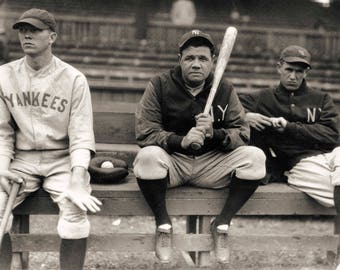In this black-and-white photograph, three New York Yankees baseball players are arranged against the backdrop of high bleachers. At the center is the legendary Babe Ruth, who is likely in the earlier part of his career given his youthful appearance. He is looking directly at the camera, gripping a bat over his shoulder while sporting a dark uniform top and light-colored pants.

To Ruth's left stands another player, also in a cap and light-colored Yankees uniform with knee-length black socks. He is holding a bat that rests on the ground, and he isn’t looking at the camera. Positioned between Babe Ruth and this player is a baseball glove with a ball nestled inside it.

On Ruth’s right sits the third player, wearing the same uniform as Ruth—dark top and light pants. He, too, looks directly at the camera but with a noticeably mean and nasty expression on his face. The image captures a moment in baseball history, emphasizing the camaraderie and uniformity of the players during that era.